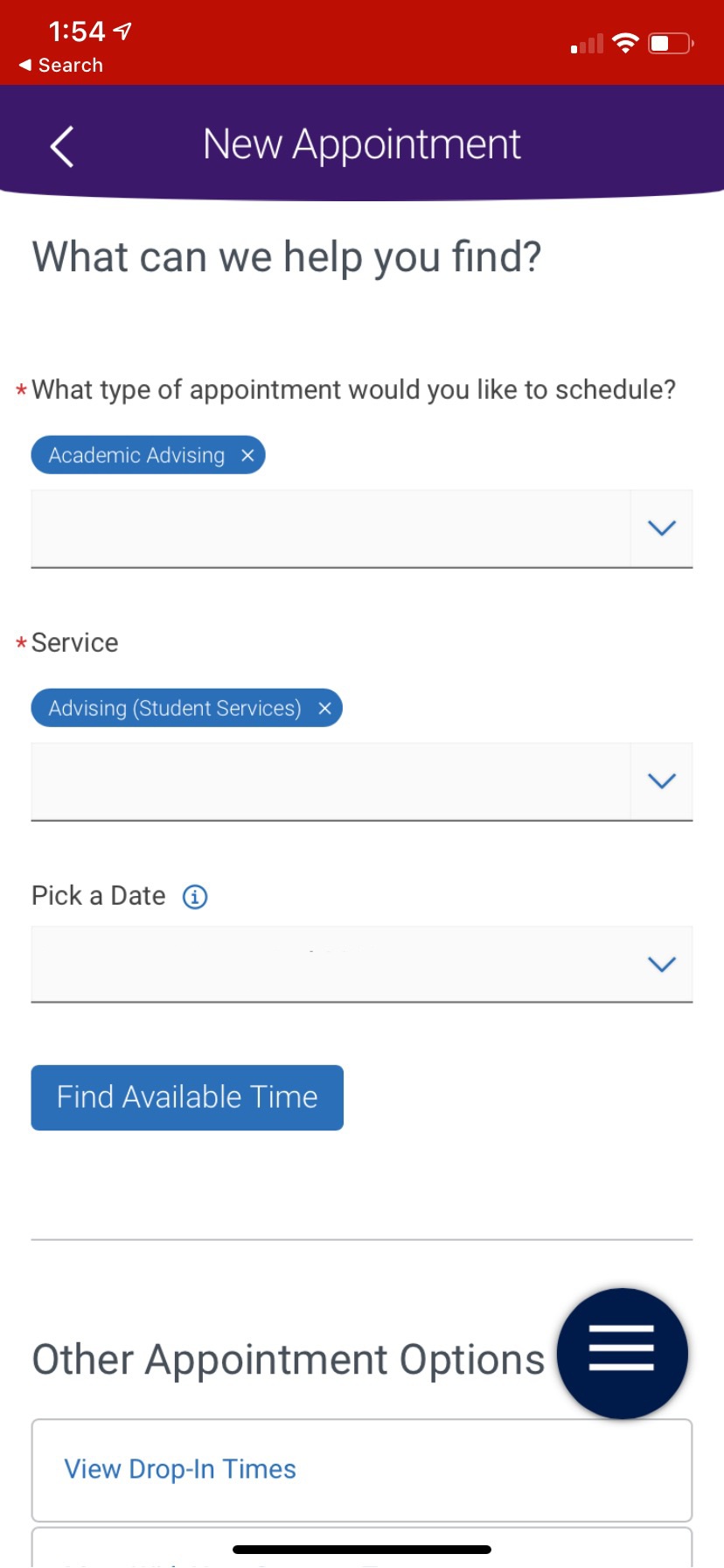This mobile screenshot captures a user interface from an application or website, likely related to scheduling appointments, with a layout characterized by distinct sections and color schemes.  

At the very top, there is a red bar housing the phone’s status icons. On the left, the time is displayed in white as "1:54" followed by a location icon. Toward the right, signal strength is indicated with one out of four bars filled, implying a weak connection. Next, there's a Wi-Fi icon indicating connectivity, and a horizontally-aligned battery icon showing a charge level around 40-50%.

Just below this, the main area features a blue background with white text reading "New Appointment" accompanied by a left-pointing arrow. Beneath this is a subheading in dark text asking, "What can we help you find?"

The next section presents a form for scheduling appointments. It starts with the prompt, "What type of appointment would you like to schedule?" labeled with a red asterisk to indicate a required field. An option for "Academic Advising" is shown as clickable white text on a blue oval background.

Further down, a text field labeled "Service" with another red asterisk appears, defaulted to "Advising Student Services" in white text on a blue oval background. Below these, an entry for "Pick a Date" includes an information icon, followed by a dropdown menu. A button labeled "Find Available Time" in white text on a blue rounded background sits at the bottom of this form section.

A horizontal line separates the form from another subheading that reads "Other Appointment Options," accompanied by a white three-row hamburger menu icon on a dark blue circle background. The final option displayed is "View Drop-in Times," enclosed within a box formation.

The organization, color contrast, and iconography suggest an intuitive design aimed at guiding the user through scheduling various types of appointments efficiently.